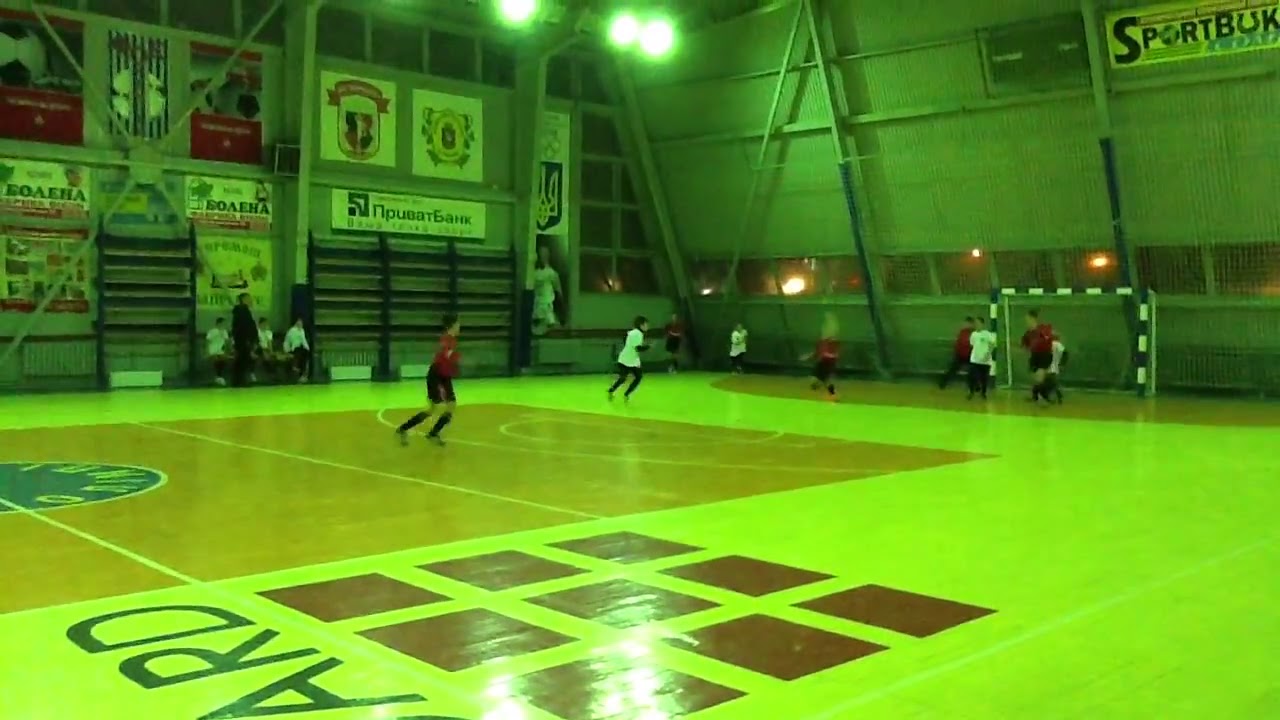A vibrant and eclectic scene unfolds in a large gymnasium lit in neon hues of green and yellow. The room, looking like it's from an indoor nighttime setting, is bustling with activity. At the heart of the action, a group of children, split into two teams wearing either white uniforms with black pants or red tops with black shorts and long socks, engage in an energetic game. The sport they're playing revolves around a goal, hinting at soccer, although a visible ball is elusive.

The gym floor is a unique blend of soccer and basketball markings, with a distinctive mix of features such as soccer goalie areas and basketball shooting zones. Prominently placed near the audience's viewpoint is a square grid composed of nine smaller dark brown squares, adorned with the letters "A-R-D" upside down to the left.

Adding to the gym's dynamic ambiance, the high walls are plastered with various posters and banners, some written in English and others in Russian. The right corner of the image showcases a sign that reads "SportBuk," with the 'O' replaced by a soccer ball and the 'U' styled as a horseshoe, presented in blue and green font. 

On the left side of the image, spectators sit on benches, observing the lively game, while the right side features the goal area where most players congregate. Various colored lights, including shades of red, blue, pink, white, and beige, contribute to the overall vivid and vibrant atmosphere of the gymnasium.